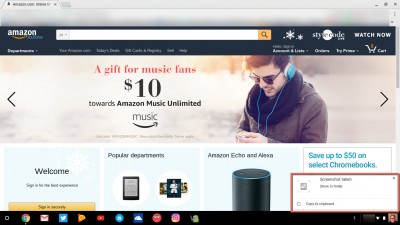This image is a screenshot of the Amazon homepage. The top portion of the page features the Amazon logo in the top left corner, alongside a long, unfilled search bar. In the top right corner, there's the text "Watch Now," followed by some blurry and unreadable text and tabs. Next to the tabs is an image of a shopping cart with a number, likely "1," though it's blurry and hard to see.

Below the header, a large banner image spans the width of the page. On the left side of the banner, there are blended colors of white and tan. On the right side, a man wearing blue headphones, sunglasses, and a thick coat is looking down. To the left of the image, bold black text reads "A gift for music fans" and below that, "$10 towards Amazon Music Unlimited." Positioned beneath this, "music" and the Amazon logo are also visible.

On the left side of the page, there's a prompt that says, "Welcome, sign in for the best experience," followed by a sign-in button. To the right of this prompt, text reads "Popular Departments," above two images resembling a tablet and possibly a phone screen. Further right, there's a section that says "Amazon Echo and Alexa" accompanied by an image of a smart speaker. Adjacent to this, there is text that reads "Save up to $50 on select Chromebooks."

The bottom of the page is bordered by a black strip.